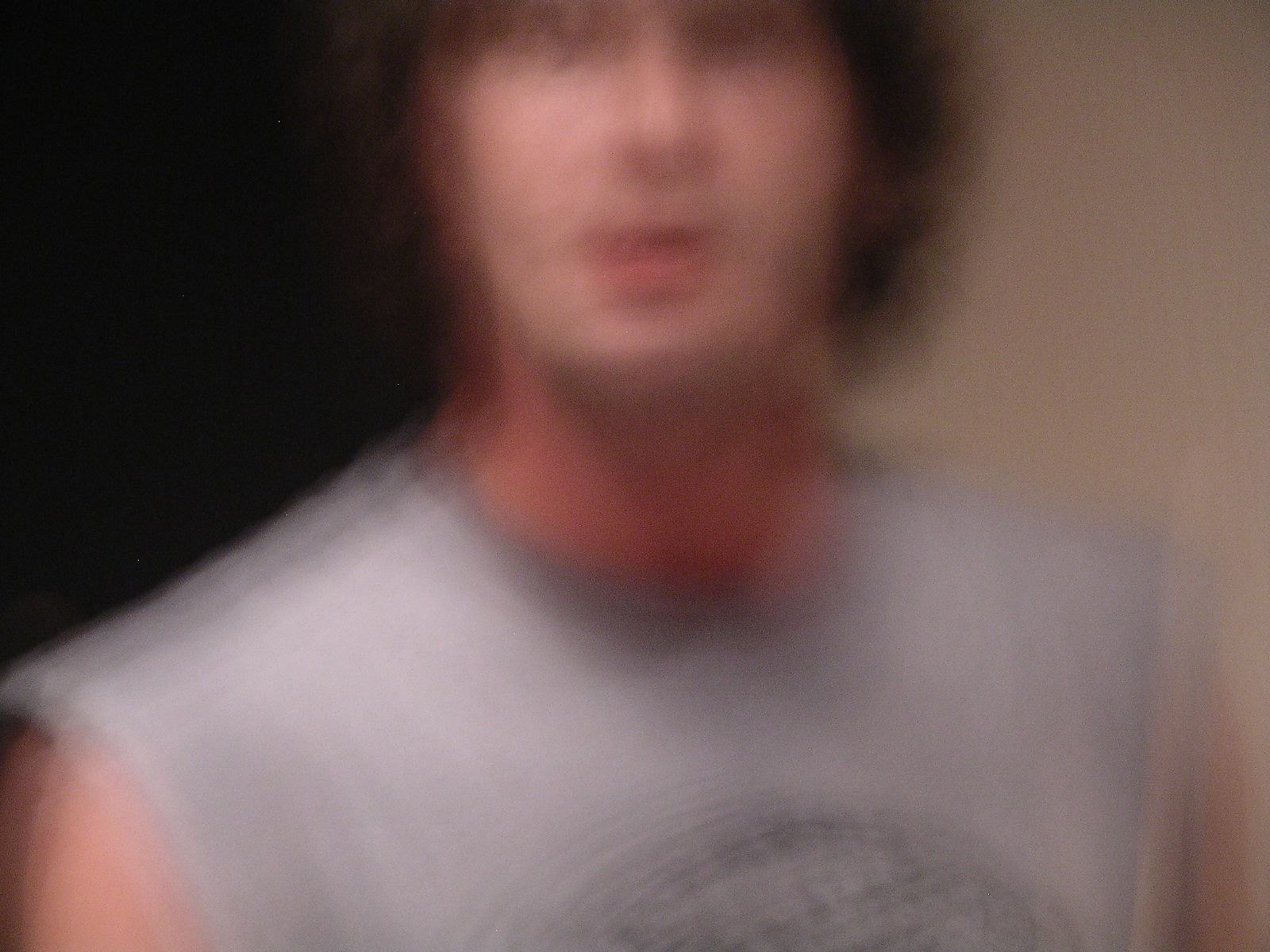The image shows a blurry photo of a male figure, featuring only the lower part of his head, neck, shoulders, and upper chest. He has short, dark brown, curly hair that is a bit puffy. He is wearing a light gray sleeveless t-shirt, darker around the collar with a possible sweat stain. The shirt has a circular or oval print with indistinct writing and a black illustration at the center, but due to the photo's blurriness, the details are unclear. The background is split, being black on the left side and tan or white on the right side, with the top left showing a shadow on the person's neck.